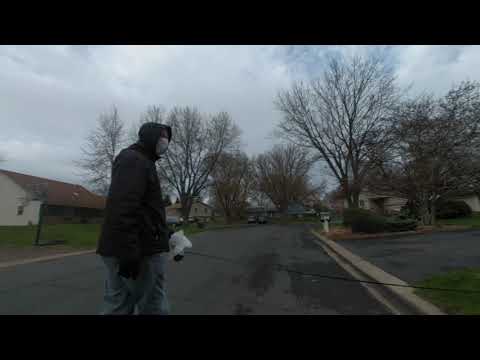This detailed photograph captures a man walking his dog in a residential neighborhood, although the dog is not visible. The man, positioned left of center and walking towards the right in a side profile, is bundled up in a black hooded winter coat, black gloves, a black jacket, and gray pants, clearly indicative of the chilly weather as the leafless trees suggest it's winter. A white surgical mask covers his face, a recognizable sign of the pandemic times. In his left hand, he holds both a leash that extends out of the frame and a bundled plastic bag, likely for picking up after his dog. The setting is a dreary, overcast day with a sky thick with clouds. The neighborhood features several houses with brown roofs and tan siding, mailboxes out front, and barren trees scattered around. To the right, there's a curb and a small parking area, while in the distance behind the man, a stone house with a brown roof and a couple of parked cars are visible, anchoring the scene of a typical, quiet residential street.